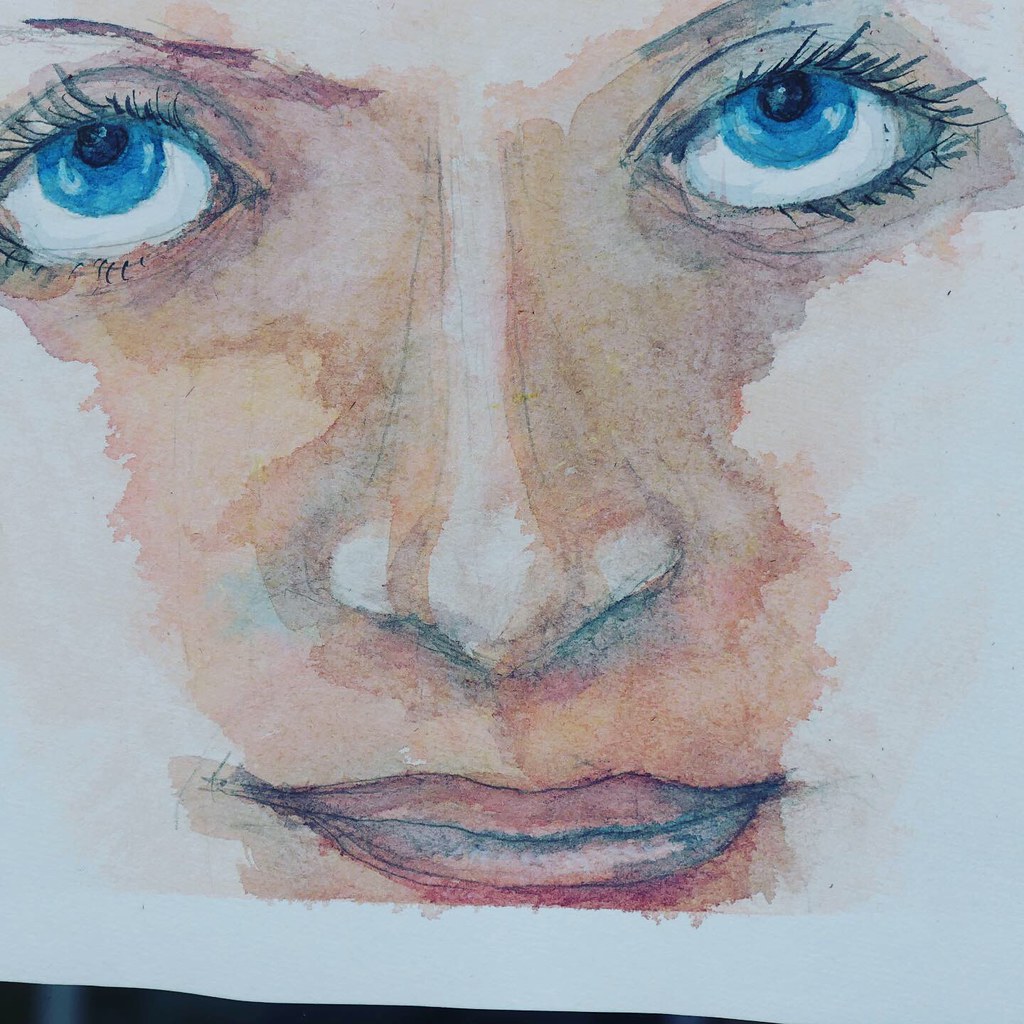The image is an extremely close-up photograph of a watercolor illustration of a woman's face in progress. The artwork, sketched and then painted, reveals construction pencil lines beneath the watercolors. The subject's facial features are detailed and prominently focused in the frame, presenting an intense, almost mesmerized expression.

The woman's blue eyes are particularly striking, looking upwards with pronounced, black mascara-coated eyelashes on both the top and bottom lids. Thin brown eyebrows frame the eyes, and the whites of the eyes are visible around the bright blue irises, enhancing the intensity of the gaze. The eyelids are also detailed in the painting.

The nose, centrally located, is lightly shaded with a mix of brown and white tones to define its shape, including fine detailing at the tip and shadowing around the nostrils and folds. The lips are thin, lightly pressed together with a horizontal separation, showcasing multiple colors. The upper lip is dark brown, while the lower lip has shades of brown, blue, and hints of red.

The image is cut off at the chin and the full outline of the face and hair is not visible. There is also a portion of the left eye slightly cropped at the edge of the image. The background includes a dark blue strip along the bottom edge, narrowing out towards the center, and the paper itself is light gray. Some shadowing is visible beyond the artwork, suggesting the photograph was not perfectly centered.